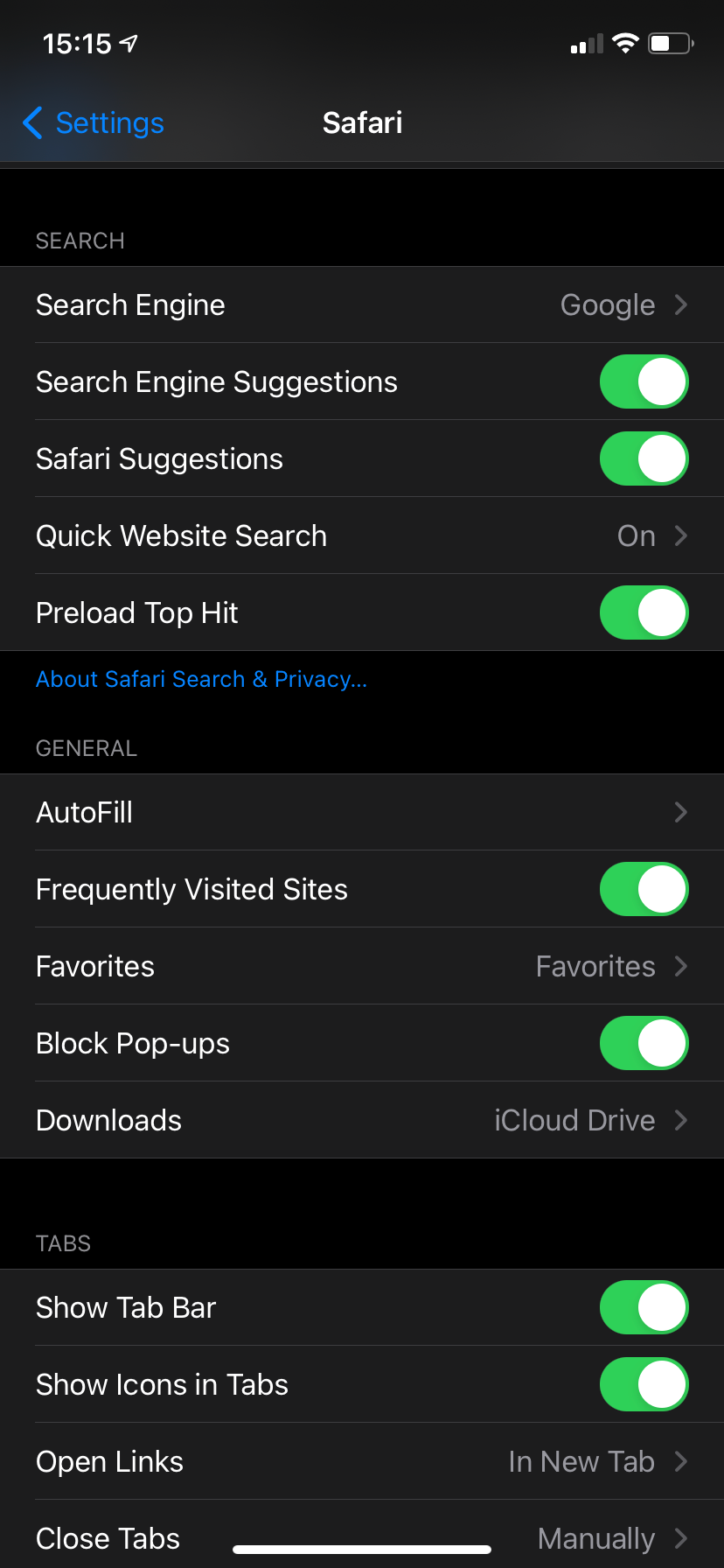The screenshot depicts a cellphone screen displaying the settings menu for the Safari browser. The background at the top is black, showing the time as 15:15, the battery life indicator, and connectivity bars. Below that, there is a blue arrow pointing left labeled "Settings," and centered in white text is the word "Safari."

In the visible settings options, the first section begins with a search bar labeled "Search," followed by toggles for various options such as "Search Engines," "Search Engine Suggestions," "Safari Suggestions," "Quick Website Search," and "Preload Top Hit," all of which are currently enabled. Directly beneath these options is a clickable blue link labeled "About Safari & Search," accompanied by an ellipsis.

Further down, under the "General" category, the screen displays options like "Autofill," "Frequently Visited Sites," "Favorites," "Block Pop-ups," and "Downloads," all of which are either turned on or have arrows indicating additional information is available. The final section is "Tabs," featuring options for "Show Tab Bar," "Show Icons in Tabs," "Open Links," and "Close Links," each of which is either enabled or has a clickable arrow for further details.